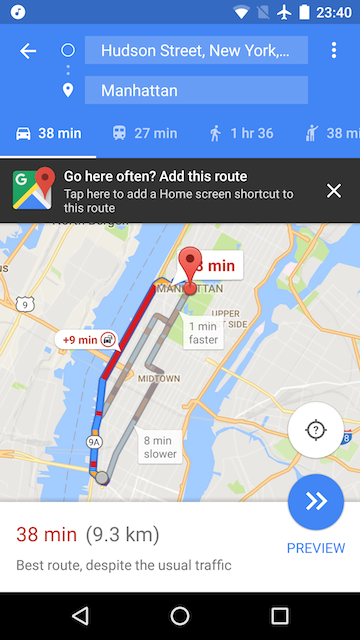This screenshot captures a detailed view of a Google Maps interface on a mobile device during a search for Hudson Street, Manhattan, New York. The top section of the screen features a light blue background with a dark blue band at the very top. Within this dark band, on the left side, there is a white circle with an emblem inside. On the right side of the dark blue band, various status indicators are visible including the Wi-Fi symbol, another status icon, airplane mode symbol, battery level, and the time, which is 23:40.

Directly below this, a lighter blue section houses navigation elements: a left arrow on the far left and three vertical dots indicating additional options on the far right. The central part of this lighter blue area contains a slightly grayed-out field for entering search criteria. 

The current search is for Hudson Street, Manhattan, New York, providing several commuting options: 38 minutes by car, 27 minutes by train, 1 hour and 36 minutes walking, or 38 minutes by cab.

Beneath this information but above the map, a black bar spans the entire width of the screen. On the left of this bar, the Google Maps logo is visible, followed by text in white reading, "Go here often? Add this route." Additional text suggests tapping to add a home screen shortcut for this route, and on the far right, there is an 'X' for closing the bar.

The map itself shows a portion of Manhattan with selectable transportation options clearly displayed. Below the map, a white block indicates the quickest route: 38 minutes, covering 9.3 kilometers. The duration is highlighted in red, while the distance is in dark gray. Beneath this, gray text mentions "Best route despite the usual traffic."

At the bottom right corner of the map, a blue circle with two right-pointing arrows in white is labeled "Preview," and above it, a white circle contains a compass symbol. The very bottom of the screenshot displays the mobile device’s black navigation bar, featuring a white triangle pointing left, a circle in the middle, and a square on the right.